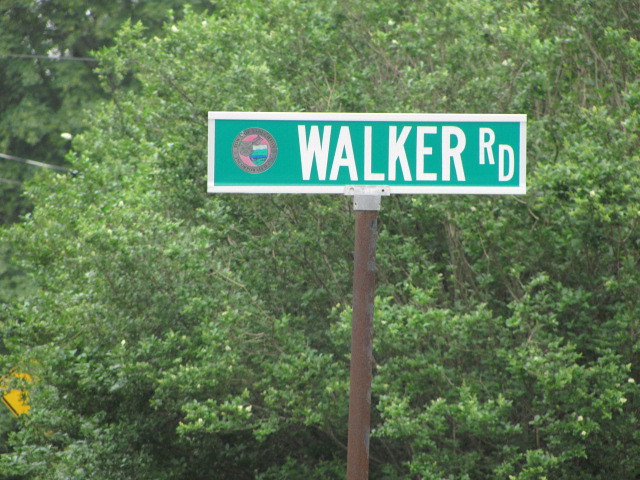The photograph captures a street sign for "Walker Road" prominently displayed on a slightly rusty, round post. Despite the rust on the post, the sign itself appears relatively new. Intriguingly, the lettering for "RD" is staggered, with "R" positioned above "D," which gives it a unique and eye-catching appearance. The text "Walker" and "RD" are both in white, set against a green background, and enclosed within a white border. In the top-left corner of the sign, there is a small emblem, though its details are too minute to discern.

In the background, a dense array of trees and foliage extends across the scene, contributing to the lush, leafy surroundings. Overhead, some power lines and communication lines traverse the upper left corner of the image. The photo seems to be taken on a sunny day, lending a bright and inviting atmosphere to the scene.